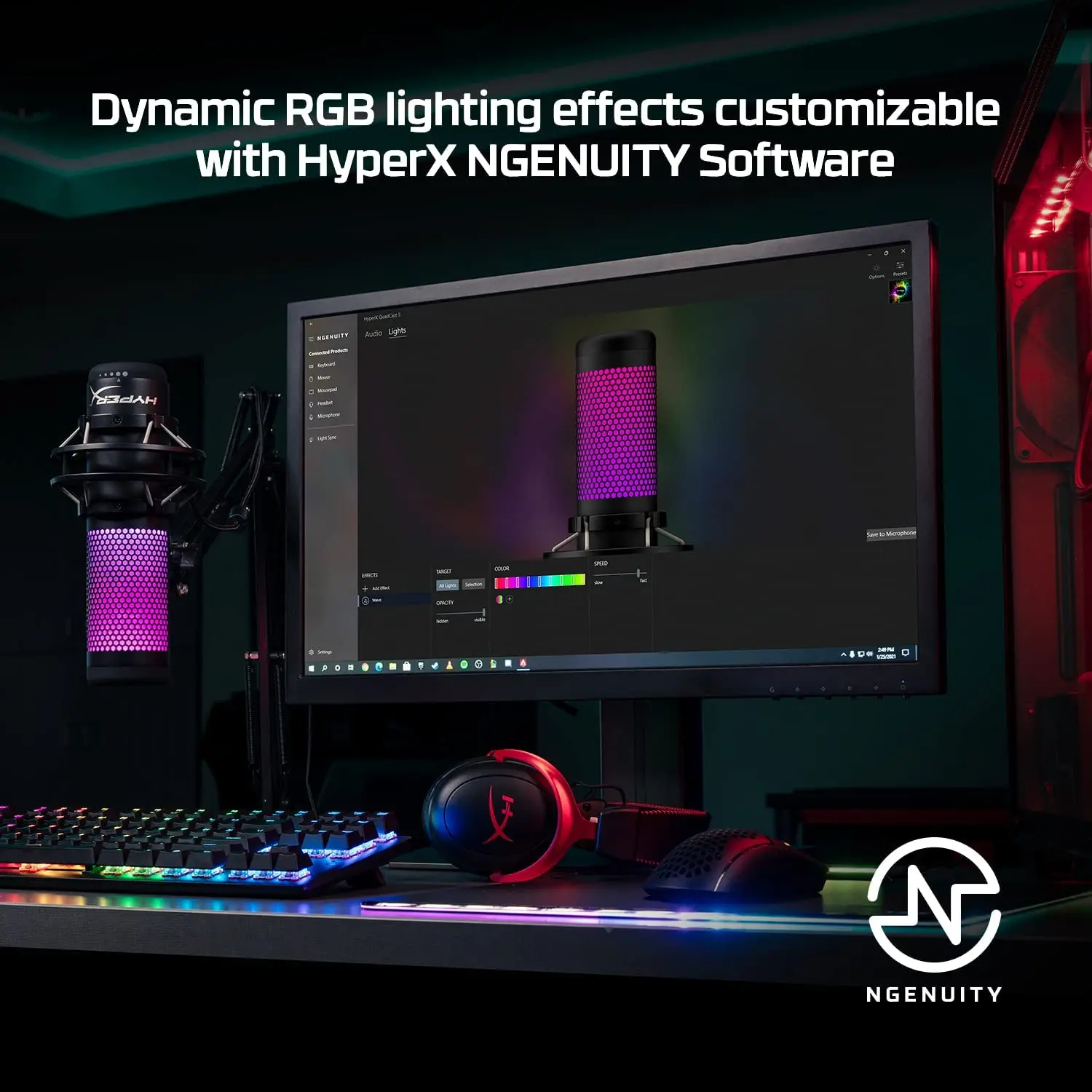This image is a sleek, square-shaped advertisement with a predominantly black background, highlighting dynamic RGB lighting effects customizable via HyperX Ngenuity software. Across the top of the image, crisp, white text reads: "Dynamic RGB lighting effects customizable with HyperX Ngenuity software." In the bottom right corner, a distinctive circle features an "N" in its center, with "Ngenuity" inscribed below it in bold white text. 

The photograph centers on a black computer desk illuminated by vivid RGB lighting. Dominating the right side is a desktop computer with red LED lights, set against the glowing background of a dimly lit room. To the left, a black microphone arm holds a cylindrical microphone glowing purple, mirroring the spectrum of colors depicted on the screen. Below this, an RGB keyboard emanates a rainbow of colors from red to blue, and to its right, a black over-the-ear headset with red accents rests. The meticulous lighting effects, accentuated by the RGB keyboard and headset, underscore the high-tech, customizable features promoted by HyperX Ngenuity software. The dark, atmospheric setting enhances the vibrant colors and high contrast, making each element of the advertisement stand out sharply.